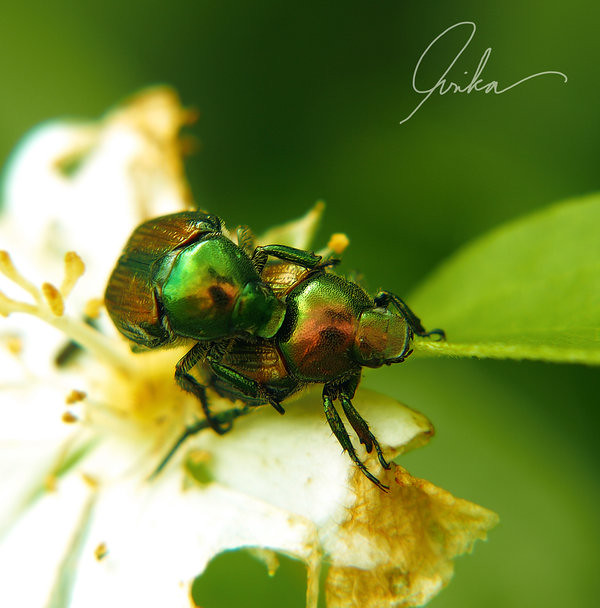In this detailed close-up image, we observe two iridescent green beetles, one perched atop the other, likely engaged in mating. Their bodies shimmer with hues of green and gold, accentuated by both green and black legs. The beetles are resting on a verdant green leaf, which is part of a plant that also features a white, slightly fuzzy flower with a hint of orange at its edges. The flower, situated mainly towards the bottom left of the frame, shows signs of damage, possibly from the beetles feeding on it. The background is out of focus, consisting mainly of blurred green shades, ensuring the insects and the flower are at the center of attention. The top right corner of the image bears a cursive watermark that appears to spell out "A-R-I-K-A."